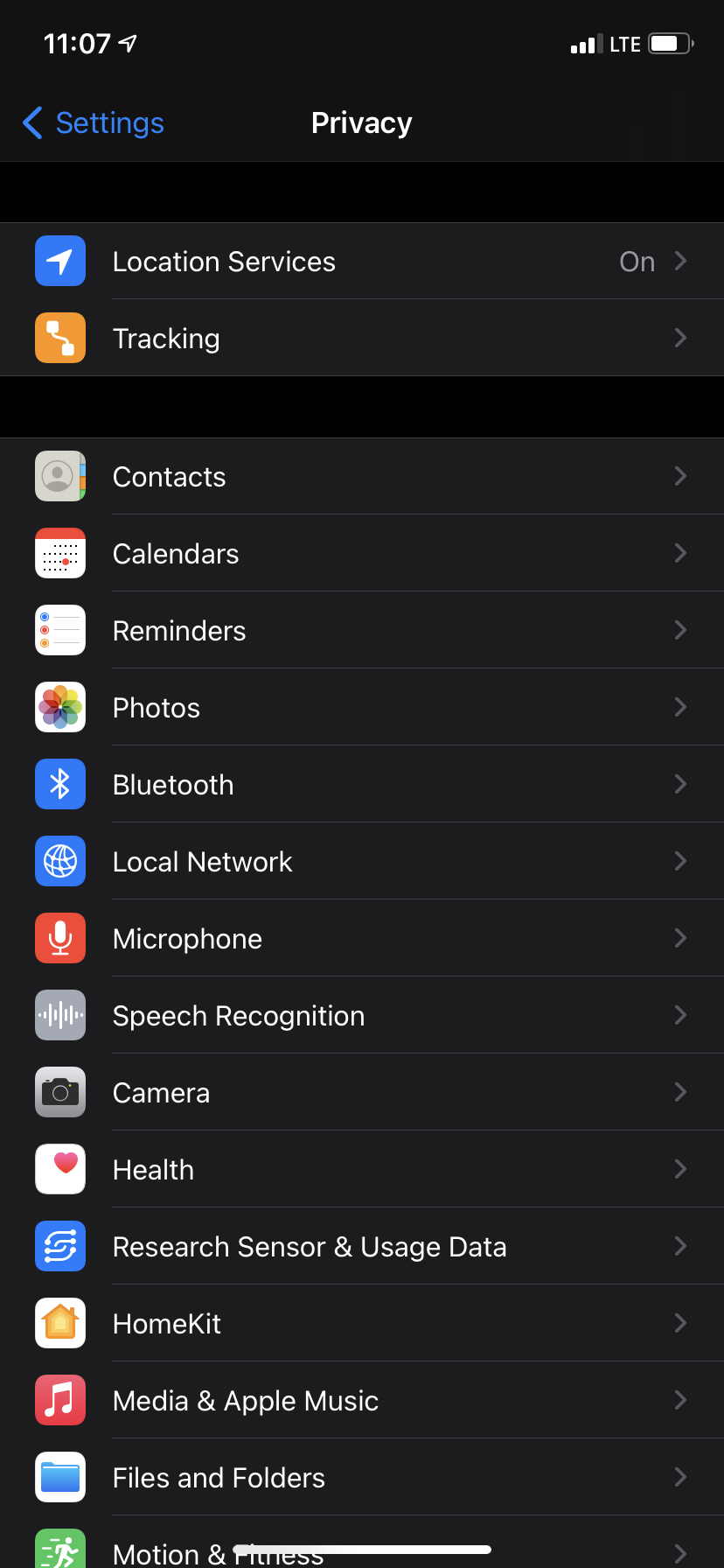This is a detailed screenshot of an iPhone settings page, focused on the Privacy section. The status bar at the top indicates the time as 11:07, displayed in white text. Directly beneath the time, the word "Privacy" is centered at the top of the screen in white text, signifying the current menu. On the left-hand side, there's a blue, left-pointing arrow labeled "Settings," indicating the previous menu.

Below this header, a series of neatly aligned, evenly spaced rectangular widgets are displayed, each corresponding to different privacy-related controls. The widgets listed include:

1. **Location Services** - The only option with additional text on the right side, indicating it is turned on.
2. **Tracking**
3. **Contacts**
4. **Calendars**
5. **Reminders**
6. **Photos**
7. **Bluetooth**
8. **Local Network**
9. **Microphone**
10. **Speech Recognition**
11. **Camera**
12. **Health**
13. **Research**
14. **Sensor & Usage Data**
15. **HomeKit**
16. **Media & Apple Music**
17. **Files and Folders**
18. **Motion & Fitness**

Each of these widgets is accompanied by a greyed-out arrow on the right-hand side. The overall background of the screenshot is white, contributing to a clean and organized appearance.